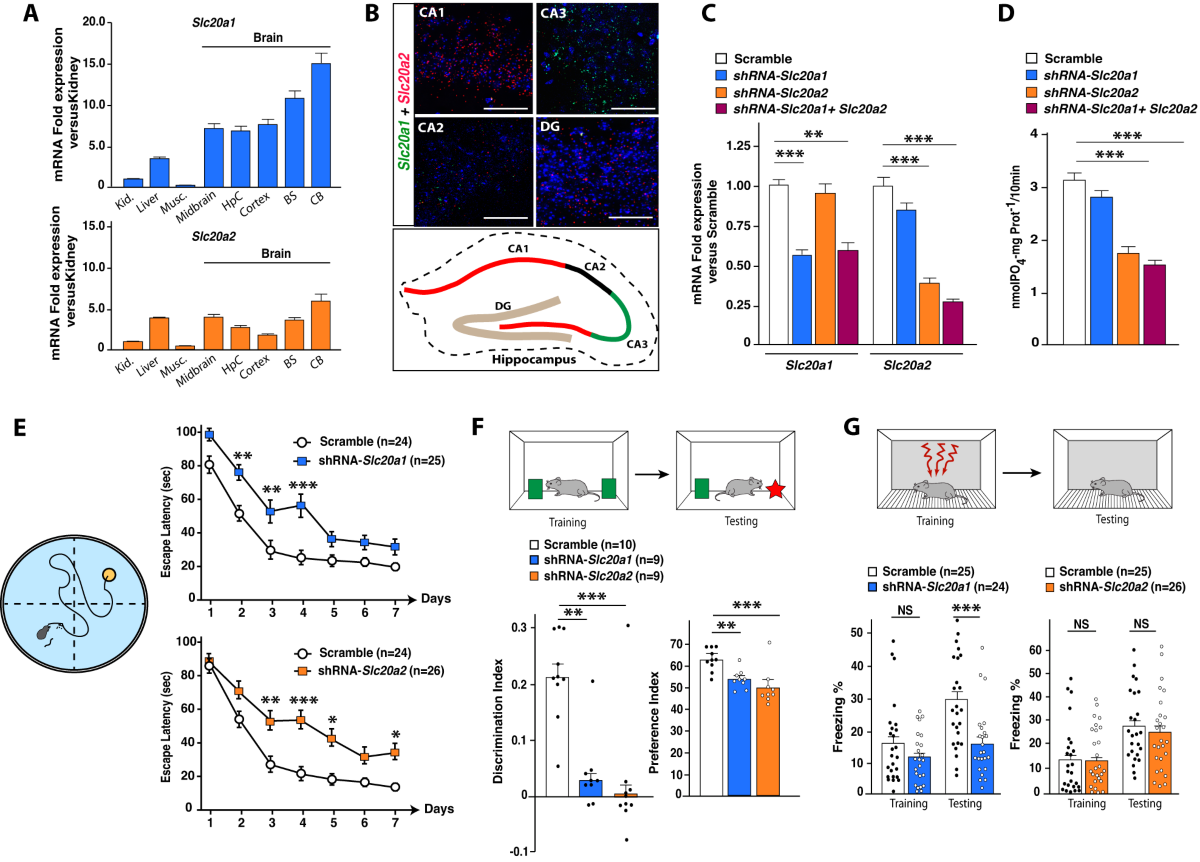This detailed image contains a series of scientific diagrams and graphs organized alphabetically from A to G, each showcasing various types of data, predominantly bar and line graphs. 

- **A**: Features two bar graphs, one in blue and the other in orange, both labeled "mRNA fold expression vs kidney," highlighting brain reactions.
- **B**: Depicts three colored images of the hippocampus, a brain region, with a focus on neural pathways.
- **C**: Presents another bar graph, labeled "mRNA fold expression vs scramble," showing similar colors to those in A and B.
- **D**: Contains an additional bar graph with no specified label.
- **E**: Includes two line graphs titled "escape latency," one in blue and one in orange, accompanied by a small image of a mouse. These graphs presumably illustrate some behavioral measure over days.
- **F and G**: Display images of mice engaged in testing and training scenarios, surrounded by blocks and stair-like structures. Additionally, these sections contain bar graphs and diagrams, where terms like "discrimination index" and "training vs testing" are observed. F specifically shows two mice with green and red blocks and directions, while G includes similar arrangements but with emphasis on training and testing.

The recurring color scheme features blue, orange, red, and occasionally black, predominantly in bar charts and visual representations of experimental setups involving lab mice. The detailed and intricate presentation appears to align with a scientific study on mRNA expression and behavioral training of mice.